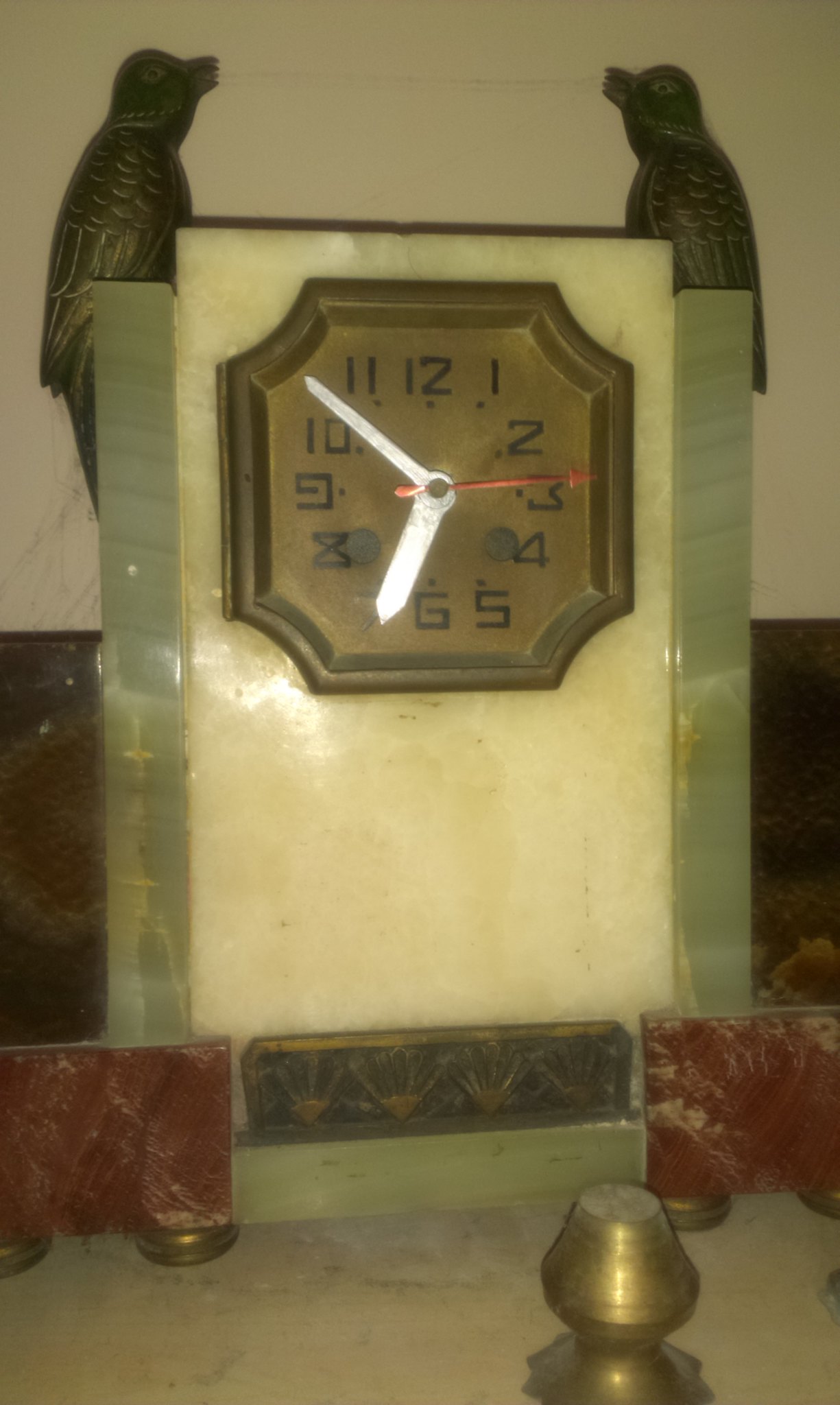The image presents a detailed composition characterized by a mix of colors and elements. The top portion of the image features a white background, seamlessly transitioning to a predominantly black bottom. In the bottom left and right corners, hints of brown are present, adding warmth to the scene. Centrally located at the very bottom is a metallic knob, which has a sloped top that broadens into a wider white base.

Anchoring the scene is a sophisticated clock positioned centrally. The clock's surface is white and possesses a reflective quality, enhancing its elegance. The clock face is unique, being segmented into four gently curving sides, each adorned with the numbers 1 through 12 arranged in a traditional clockwise sequence. The second hand is pointing right, while the hour hand is directed towards the bottom left, situated between the numbers 6 and 7. The minute hand is positioned between the 10 and 11 o'clock marks.

To the top left and right of the clock, two wing-like figures are displayed, possibly symbolizing motion or time's fleeting nature. In the left area of the image, near the clock, a large grey rectangle provides a stark contrast, framing the artwork with a modern, minimalist touch. The detailed juxtaposition of colors and elements creates a visually intriguing and balanced composition.